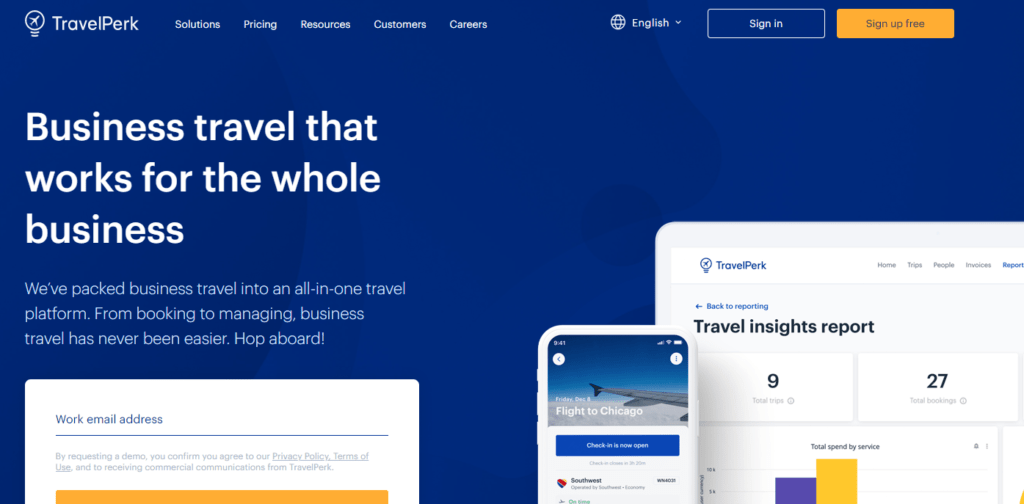In this visually engaging image, the background is predominantly blue. At the top left corner, there is a circle containing an airplane icon, next to which the text "TravelPerk" is displayed. Moving across the top line from left to right, you'll find navigation options labeled "Solutions," "Pricing," "Resources," "Customers," and "Careers." Further along, there is a globe icon with the word "English" beside it, indicating a language selection dropdown menu. 

Adjacent to this, two rectangular buttons are prominently featured: the "Sign In" button in a standard design, and the "Sign Up Free" button highlighted in orange.

On the left side of the main content area, white text reads, "Business Travel that works for the whole business." Smaller white text below elaborates, stating, "We've packed Business Travel into an all-in-one travel platform from booking to managing. Business Travel has never been easier, hop aboard."

At the top of a white, square-ish section, blue text prompts for a "Work Email Address" with an underline below it. Beneath this, there are two lines of smaller, light gray, hard-to-read text. You can also make out part of a yellow shape near the bottom left of this section, though it's partially cut off.

To the right, an image of a mobile phone displays a screen showing a scenic view of a plane wing against a backdrop of sky and clouds, labeled "Flight to Chicago." A blue button is visible but not legible. Below this, potential flight listings are indicated with the mention of "Southwest."

Partially behind the phone and in the bottom right corner of the image, another white section features the "TravelPerk" logo again. This section contains various text elements and visuals related to travel insights, including phrases like "Travel Insights Report" and several numerical and graphical elements such as "9" and "27," and a bar graph with purple and yellow segments. However, some portions of this section are cut off from view.